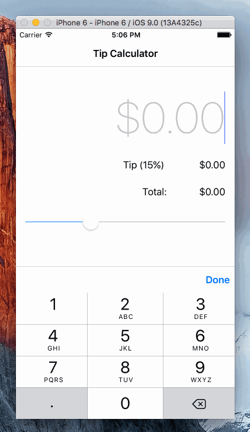**Detailed Caption:**

This image showcases an iPhone screen with an app displayed in portrait orientation. The photo is set against a blurred background that seems to depict a mountain, although the details are obscured by a central white box displaying the app interface. 

At the top of the box, there is a horizontal gray bar with three circles on the left. The first and third circles are hollow, while the middle circle is illuminated in yellow. To the right of these circles, the text "iPhone 6 - iPhone 6 / iOS 9.0 (13A4325C)" is displayed in black font, indicating the device and iOS version. 

Below this, the status bar shows the word "Carrier," a fully filled Wi-Fi signal icon, the time "5:06 p.m.," and a fully charged battery icon. 

The main interface below this section features the header "Tip Calculator" in black text, followed by a horizontal line. Beneath the line is a numerical display currently showing "0," where input can be added. Further down, the app specifies a "Tip 15%" indicator, showing "$0.00" for both the tip and the total, signifying that no values have been entered yet. 

This app evidently helps users easily calculate the tip amount for a bill and the total sum to be paid, combining the principal amount and the tip.